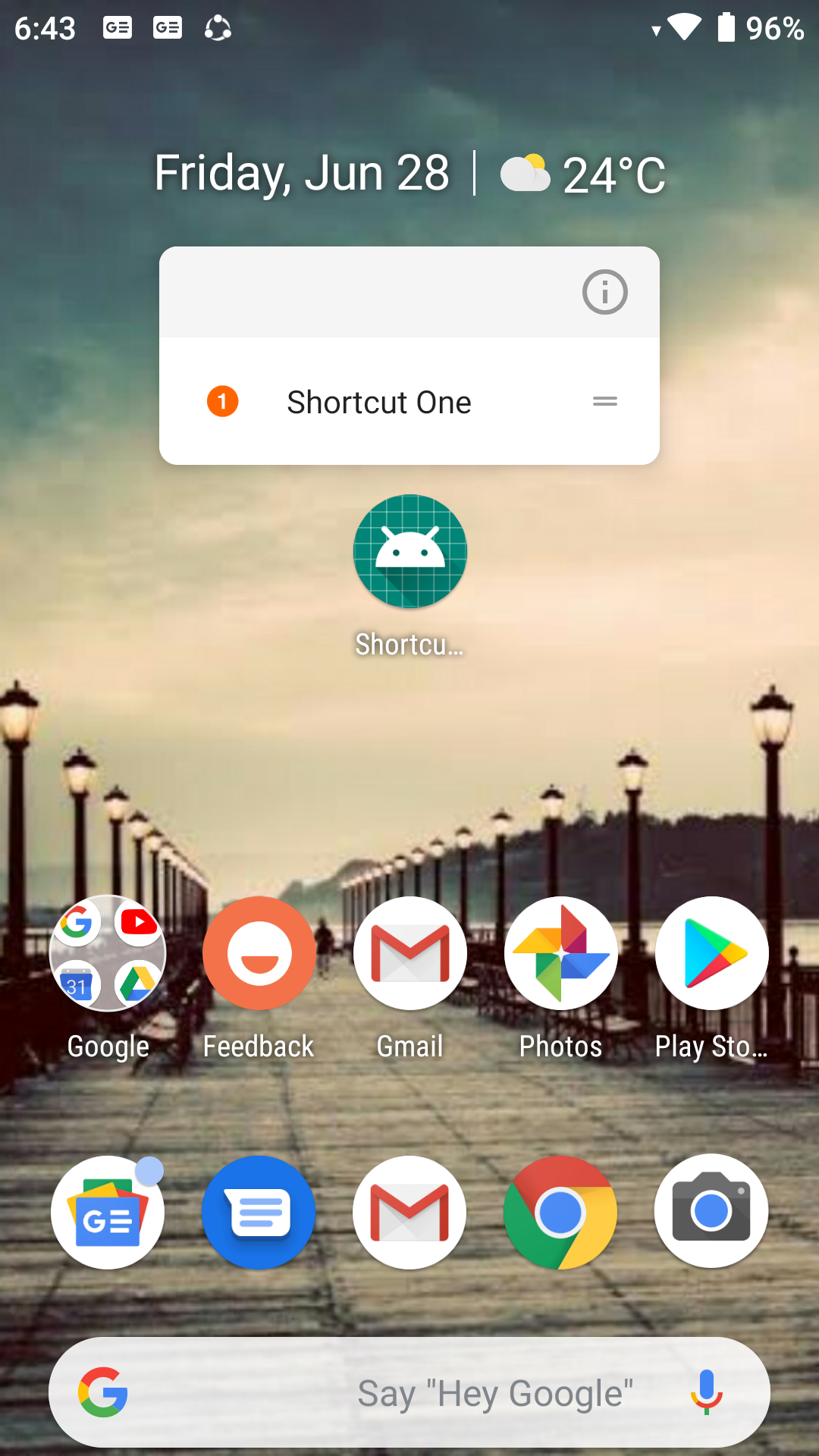This image is a screenshot from an Android device, likely a phone or possibly a tablet, showcasing the home screen. The background wallpaper features a scenic view of an old, weathered wooden pier extending into the distance under a tumultuous, overcast sky. The atmosphere is heavy with impending storm clouds, painted in shades of gray and dark green, creating a nearly monochromatic effect. Lining the pier on both sides are antique-style electric light posts, adding to the vintage charm of the scene.

The screen displays the date as Friday, June 28th and the temperature as 24 degrees Celsius, courtesy of a weather widget. A large gray rectangle, labeled "Shortcut 1," occupies part of the screen, indicating an unassigned shortcut widget. At the bottom of the screen, a Google search bar is prominently featured. Surrounding it are several circular app icons, part of the Google suite, which include Gmail, Google Chrome, Camera, Google Play Store, and Photos.